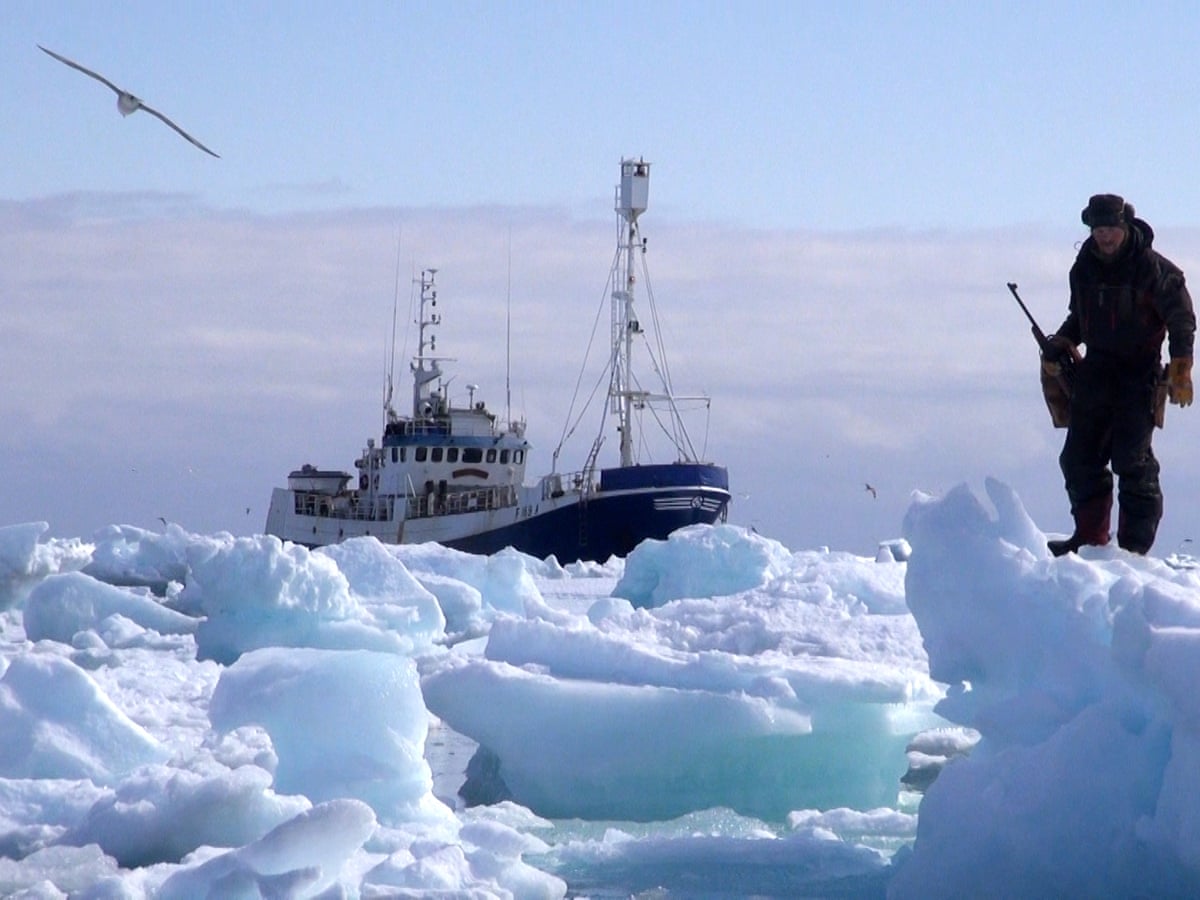In a stark, snowy environment, a large ship, primarily blue with notable black and white elements, looms in the background. The vessel appears trapped amidst the sprawling sea of ice and snow, meandering across hues of white, grey, and pale blue. Underneath pinkish-gray clouds mingling with patches of bright blue sky, a seagull soars in the upper left corner. Central to the right side of the image, a man dressed entirely in black winter clothing, including a hat, stands on the ice. He holds an unidentified object, possibly a shovel or a spear, as he gazes toward the stranded ship. The scene, brightly lit by daylight, captures the essence of a cold, isolated winter landscape, with the intricate details of the ship's towers and the mixed textures of the icy surroundings adding depth to the dramatic tableau.